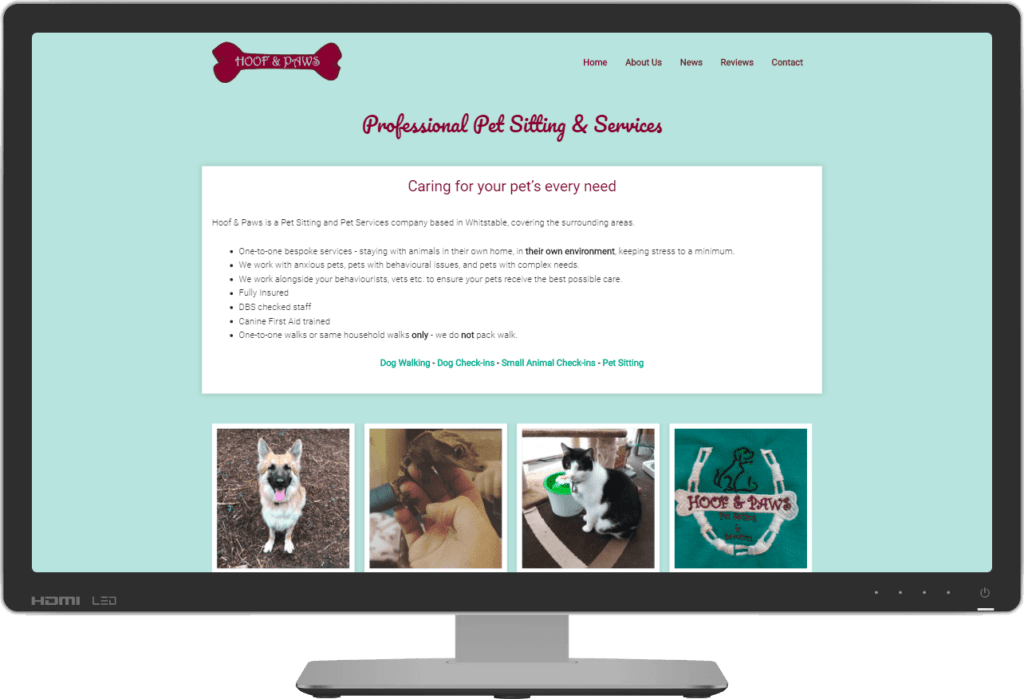The image displays the homepage of a website called "Hoof and Paws," identifiable by its logo located in the top left corner. The logo features a burgundy-colored dog bone with the text "Hoof and Paws" prominently displayed in the center in a bluish-white hue. The homepage headline reads, "Professional Pet Sitting and Services," with a subheading in a box stating, "Caring for your pet's every need."

Hoof and Paws is described as a pet sitting and pet services company based in Wistobul, servicing the surrounding areas. The page highlights a list of services they offer, including:

- One-to-one bespoke services
- Staying with animals in their own homes to keep their stress levels to a minimum
- Specializing in working with anxious pets, pets with behavioral issues, and pets with complex needs
- Collaborating with behaviorists and vets to ensure the best care
- Fully insured and background-checked staff
- Canine first-aid trained personnel
- Offering one-to-one walks or walks for pets from the same household only (explicitly stating that they do not provide pack walks)

The page also features several images, including pictures of dogs and caregivers interacting with them, as well as some branded clothing featuring the Hoof and Paws logo.